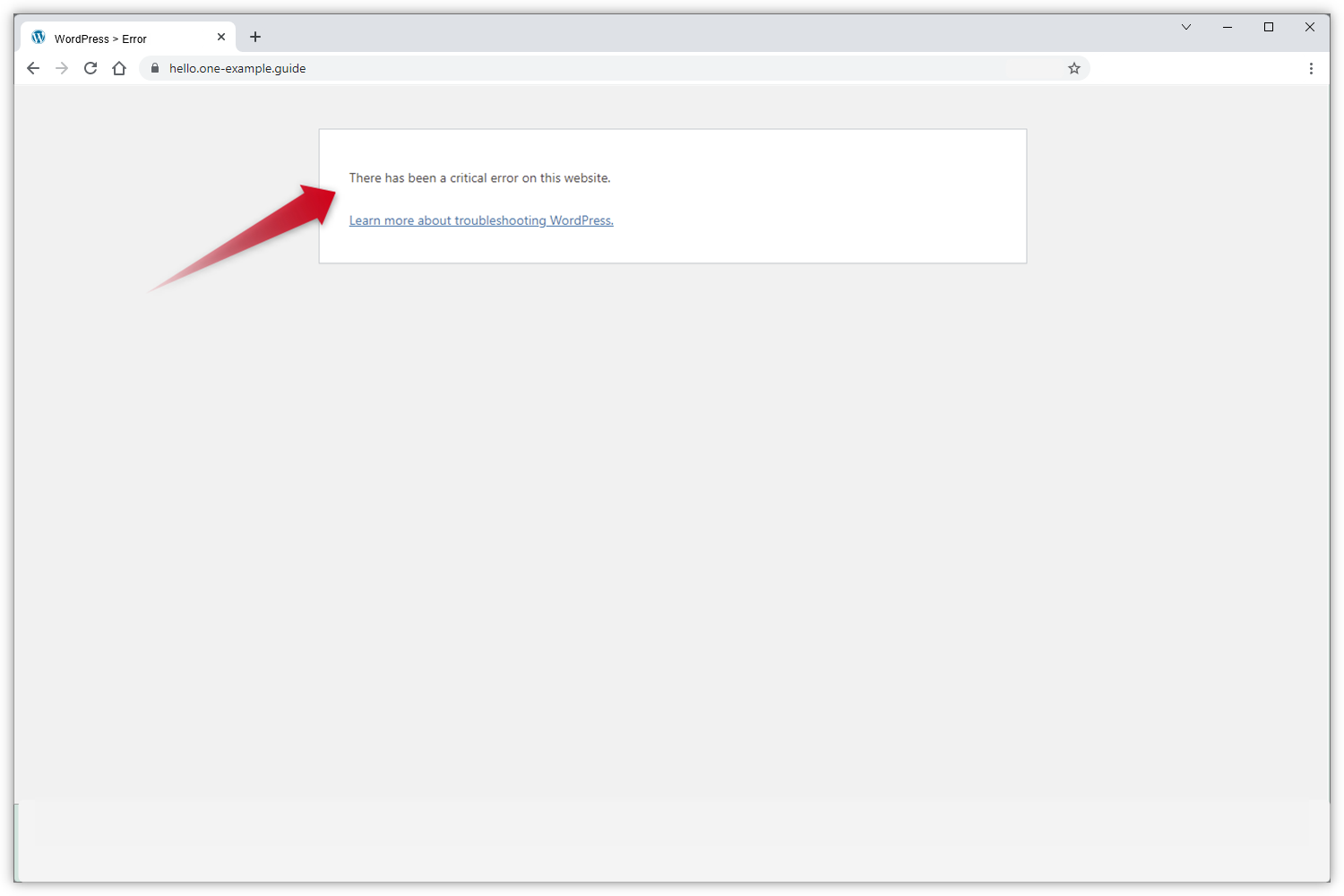Caption: 

"Screenshot of a Spring Cloud Reweb page displaying a WordPress critical error. The browser interface shows common navigation buttons such as back, forward, refresh, and home. The URL 'hello1example.guide' is visible, with tabs available for expansion at the top. On the right-hand side, there is a favoriting option. The menu buttons include minimize, maximize, exit, and an unexplained down arrow. Centrally, a white box with a gray background and a red arrow pointing towards it states, 'There has been a critical error on this website,' accompanied by a link in blue text offering to 'Learn more about troubleshooting WordPress.' The entire image captures a typical WordPress error landing page."